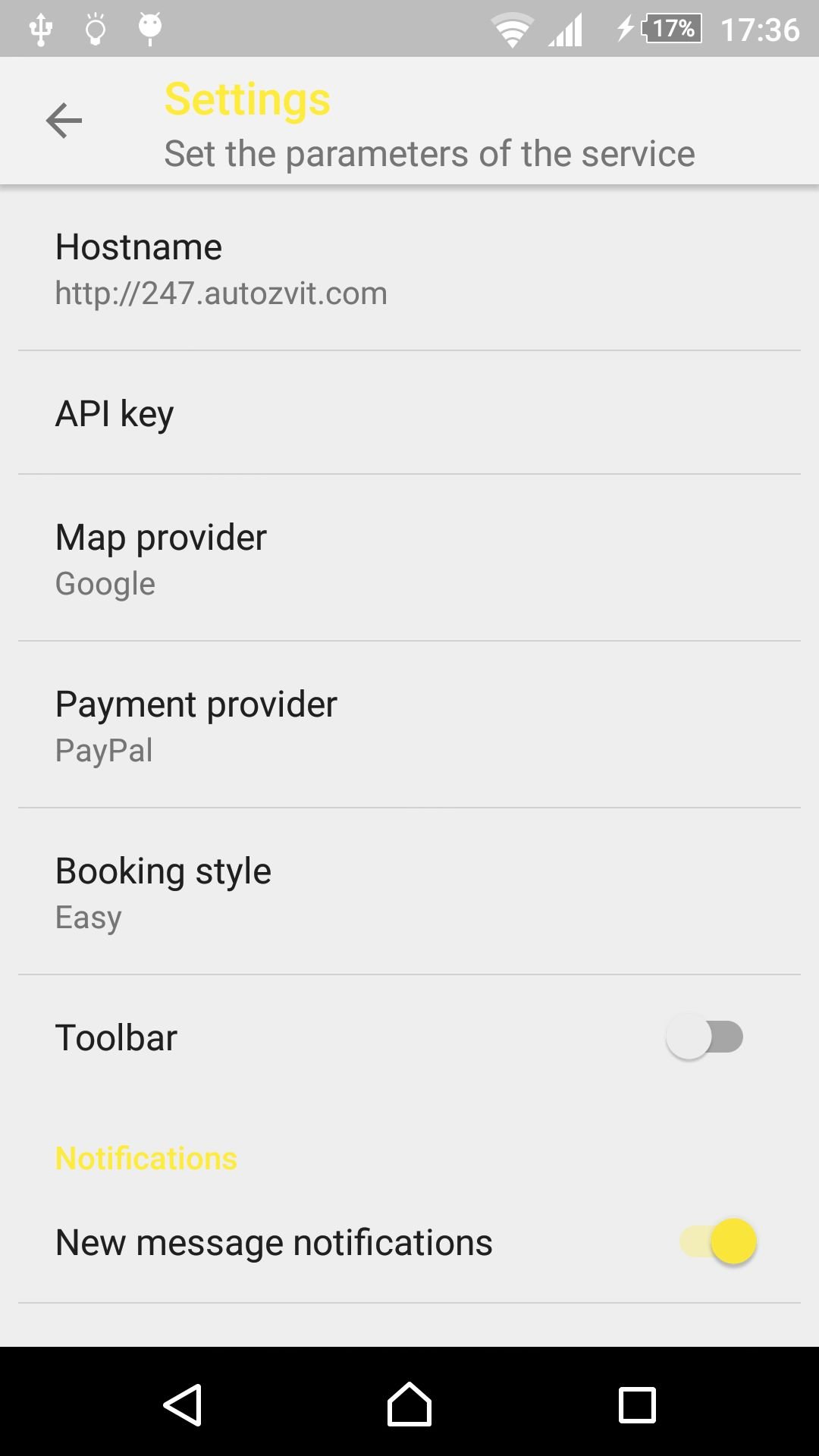This is a detailed caption for the provided image description:

*The screenshot appears to be from a smartphone interface, featuring a gray background. At the top, a gray status bar displays a strong Wi-Fi signal (4 out of 5 bars) and a battery level at 17%, shown in military time as 17:36 (5:36 PM). Below the status bar, the heading "Settings" is highlighted in yellow, followed by the instruction "Set the parameters of the service." An arrow indicating the back button is situated next to the heading.*

*The screen is divided into six rows for setting configurations:*
1. **Hostname**: http://247.autosvit.com
2. **API Key**
3. **Map Provider**: Google
4. **Payment Provider**: PayPal
5. **Booking Style**: Easy
6. **Toolbar**: Includes an on/off toggle switch (currently off).

*Below these settings, another section labeled "Notifications" in yellow includes options for new message notifications, marked as active and indicated by a yellow toggle. At the very bottom of the screen, there are several navigation icons.*